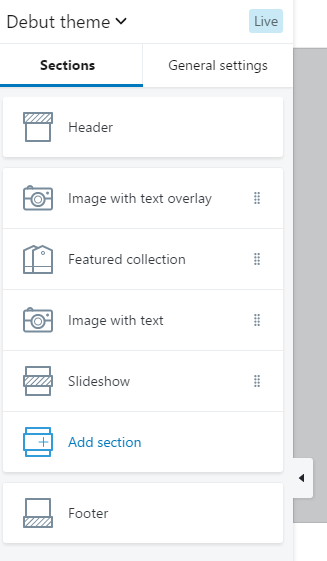The image is a screenshot from either a web or mobile device interface, showing a cropped section of a web application. The main visible element is a white rectangle, with a faint grey rectangle in the background. At the top of this section, the title "Debut Theme" is displayed alongside a black downward-facing arrow. In the top right corner, there is a blue rectangular box with the word "Live" inside it. 

At the top of the interface, there are two navigation filter buttons: "Sections" and "General Settings". The "Sections" tab is selected and highlighted by a bold blue line beneath it. Below this, there is a list of functionalities that resemble options typically found in a website builder, where you can drag and drop different elements. The functionalities listed include "Header," "Image with Text Overlay," "Featured Collection," "Image with Text," "Slideshow," "Ad Section," and "Footer," each accompanied by small icons on the left-hand side.